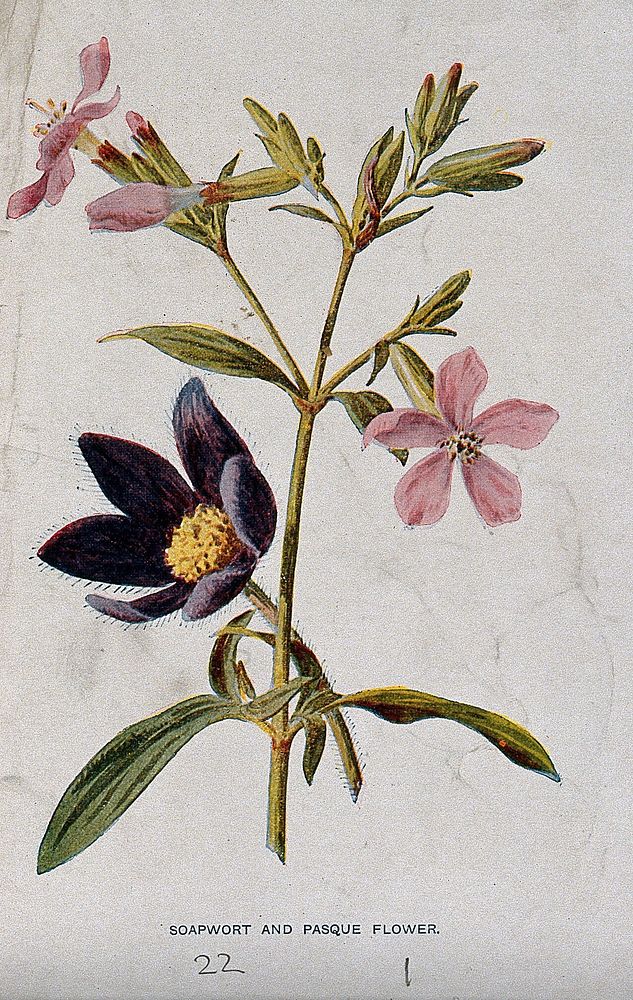The image is a detailed scanned illustration of two distinct plants with a whitish-gray, slightly grainy background, reminiscent of old paper. Dominating the foreground is a plant with a long, thin green stem bearing multiple flowers and buds. The most striking features are three pink flowers, two of which are fully bloomed with delicate pink petals and yellow centers; one is located in the upper left corner and another in the middle right. A third pink flower is just beginning to bloom in the top left corner, alongside additional buds that have not yet opened. Intriguingly, another stem, also green, supports a unique black flower with a distinctive yellow center, surrounded by small prickles protruding from both the stem and the flower itself. Below this intricate botanical illustration, the text "Soapwort and Pasqueflower" is handwritten, flanked by the numbers "22" on the left and right sides, adding to the vintage feel of the piece.